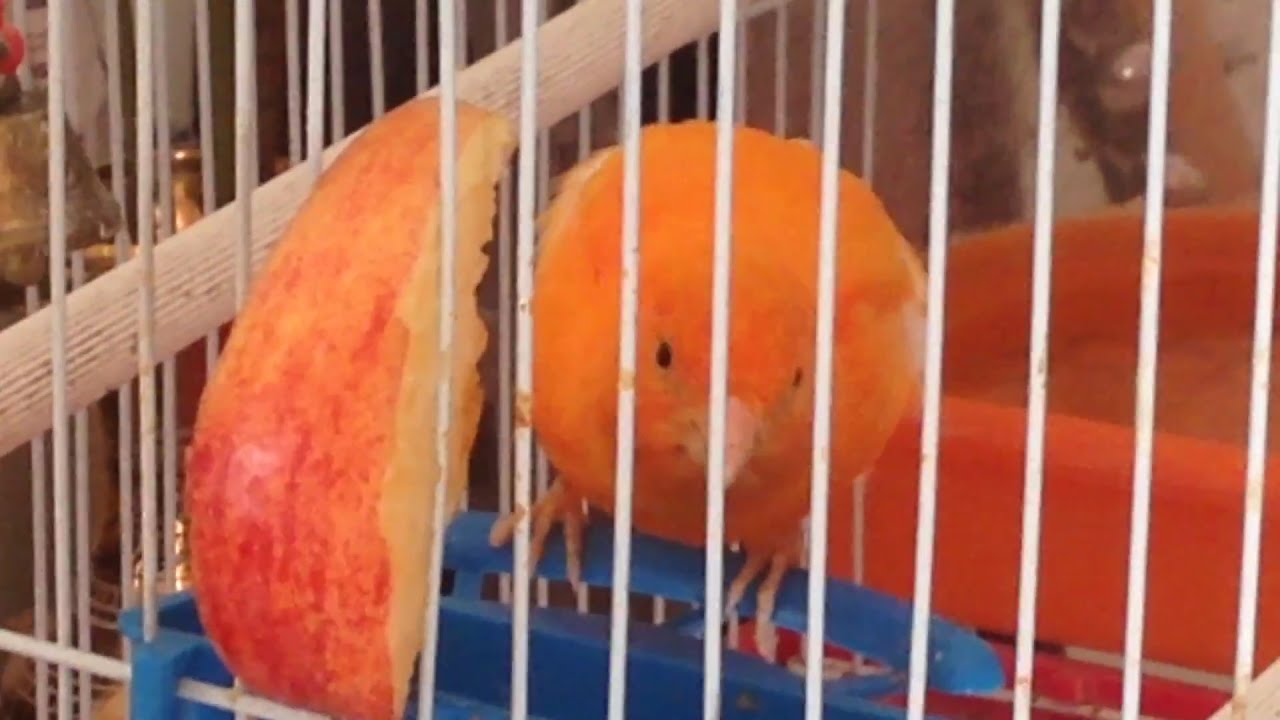The image is a detailed color photograph of an orange parakeet perched inside a white wire birdcage. The bird, which has little black eyes, a pink beak, and pink feet, appears quite plump and cylindrical, almost puffed up. It is perched on a blue plastic stand that is part of a food tray. An apple wedge protrudes through the white cylindrical bars of the cage, likely pecked at by the bird. Above the bird, there is a wooden perch, providing another resting spot. The bird's gaze is directed towards the camera, creating the impression that it is staring directly at the viewer. In the background, an orange container is visible, possibly a water bowl, and the setting suggests that the birdcage is situated within a home or apartment, as evidenced by the indistinct household items partially visible in the backdrop. The representation is highly realistic, emphasizing the photographic detail of both the bird and its surroundings.